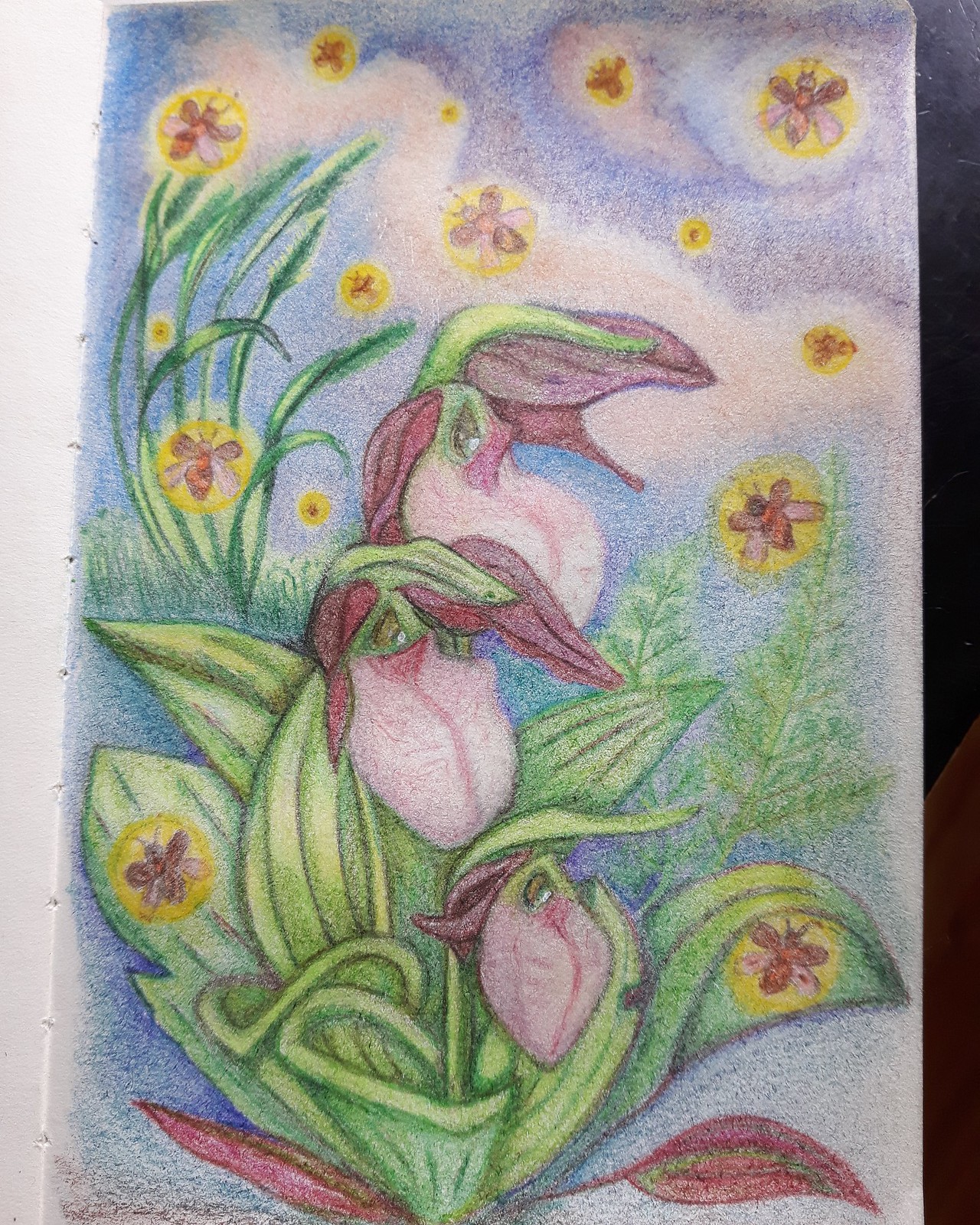This photograph showcases a captivating piece of artwork meticulously drawn on a sketch pad, likely using colored pencils, though it might also be paint. The centerpiece of this artwork is a unique and fascinating flower, boasting a large green body adorned with flat green leaves. The main flowering structure features prominent, sizable blossoms with vibrant pink petals gracefully hanging down, while striking burgundy petals rise above them, creating a striking contrast. The background is artfully rendered to depict a serene white and blue sky, enhancing the overall composition. The image is free of any text, allowing the viewer to fully appreciate the intricate details and color harmony of the artwork.